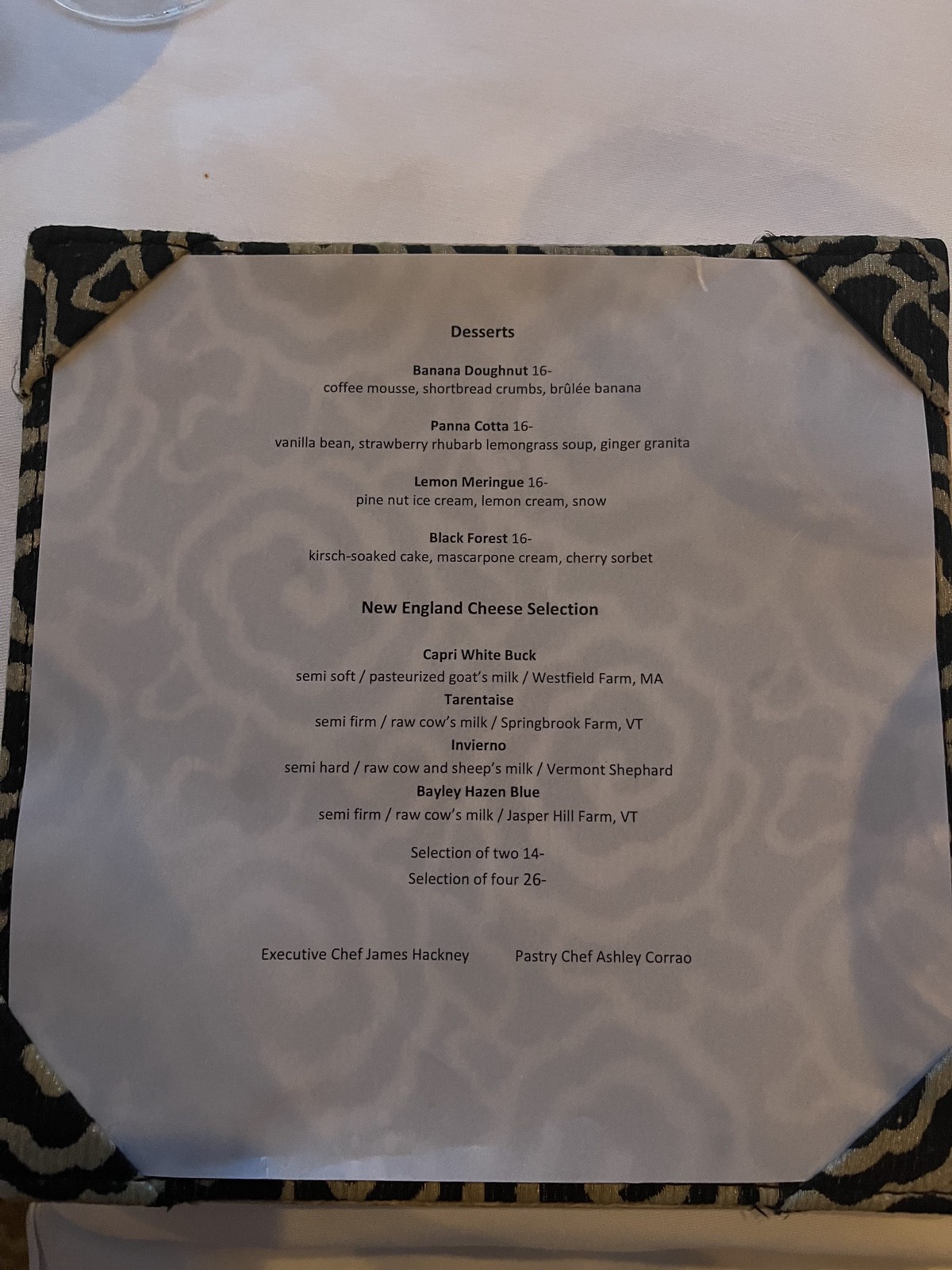The menu photograph shows a meticulously designed back cover made of black fabric, adorned with tan lines resembling animal-like spots and stripes. The white paper inside the menu allows some of these fabric patterns to subtly come through. The menu features the following detailed dessert listings:

### Desserts

1. **Banana Donut - $16**
   - Coffee mousse
   - Shortbread crumbs
   - Brulee banana

2. **Panna Cotta - $16**
   - Vanilla bean
   - Strawberry rhubarb and lemongrass soup
   - Ginger granita

3. **Lemon Meringue - $16**
   - Pine nut ice cream
   - Lemon cream
   - Snow

4. **Black Forest - $16**
   - Kirsch-soaked cake
   - Mascarpone cream
   - Cherry sorbet

5. **New England Cheese Selection**
   - Capri White Buck: Semi-soft, pasteurized goat's milk from Westfield Farm, MA
   - Tarentaise: Semi-firm, raw cow's milk from Springbrook Farm, VT
   - Invierno (additional types listed in 5 more lines beneath)

At the bottom of the menu, it notes the executive chefs responsible for these delicious offerings:
- Executive Chef James Hackney
- Pastry Chef Ashley Corrao